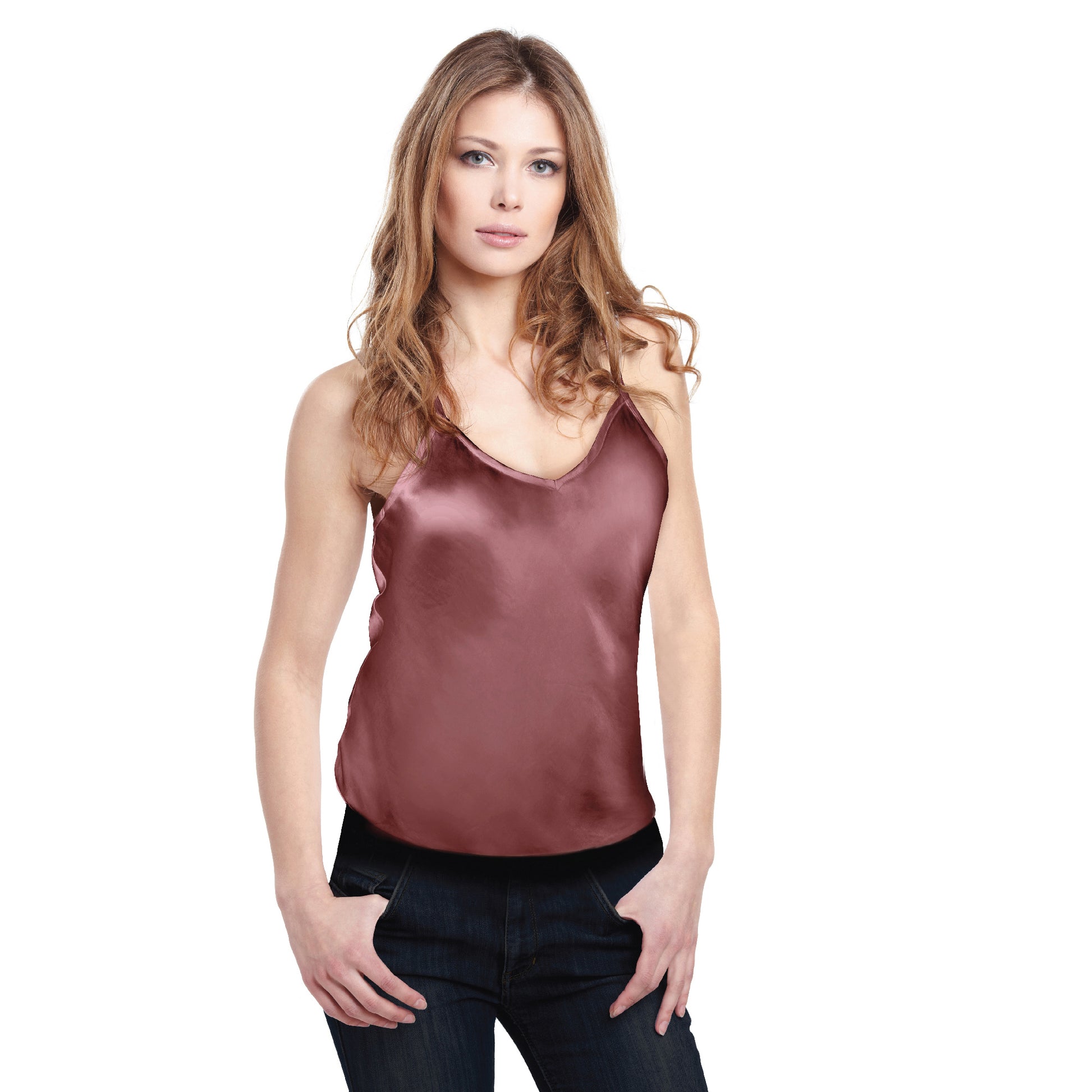The image features a woman standing directly in the middle, facing the viewer with her dark eyes making direct eye contact. She has long, reddish-brown hair that is straight with curls at the ends, parted down the middle and cascading over her shoulders. Her eyebrows are brown, and she has full, pink lips slightly parted, revealing just the edges of her teeth. She wears a satiny, light burgundy tank top, which complements the rich tones of her hair and skin. Her arms hang naturally at her sides, with thumbs hooked into the front pockets of her dark blue jeans. The photo captures her from the middle of her thighs upwards. There is a light, neutral background that highlights her figure prominently, devoid of additional text or objects.